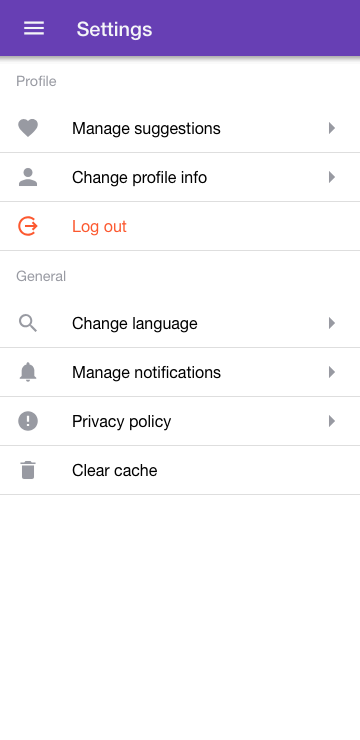In the image, we see the settings menu of an application displayed prominently. The interface features a clean design with a white background and black text. At the top, a purple header bar labeled "Settings" is accompanied by a three-line icon, commonly representing menu options. Below this header, the main content of the page begins with the word "Profile" followed by several distinct sections.

There are seven clickable sections within this page:
1. **Profile**: This section includes "Manage Suggestion Settings" illustrated with a heart icon, "Change Profile Info" marked by a person icon, and a "Logout" option, which is highlighted in either orange or red for emphasis.
2. **General**: This broader section includes:
    - "Change Language" with a magnifying glass icon.
    - "Manage Notification" with a bell icon.
    - "Privacy Policy" with a circle containing an exclamation mark.
    - "Clear Cache" identified by a trash can icon.

Each section and option is designed to facilitate user interactions with common settings tasks such as changing language preferences, managing notifications, reviewing privacy policies, and clearing cached data. This structured layout provides users a straightforward way to navigate and customize their application experience.